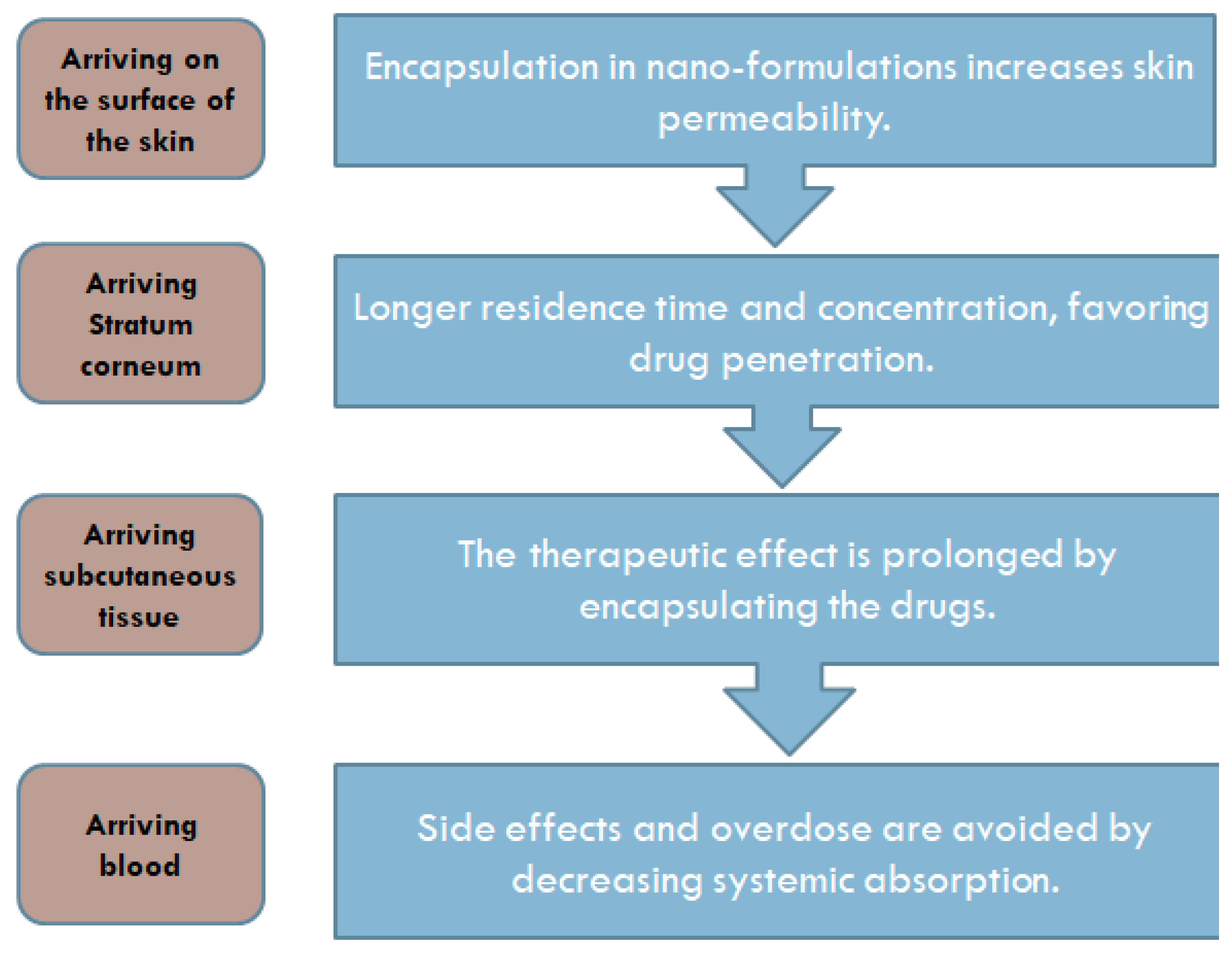This image is a detailed educational diagram, typically found in a textbook, that illustrates the process of drug delivery through the skin in a stepwise manner. The background is white, with the information presented in two parallel columns. 

The left column has small tan or peach boxes with black text, while the right column features larger light blue rectangles with white text and downward-pointing arrows connecting each step. 

At the top of the left column, the box reads "Arriving on the surface of the skin," corresponding to the blue rectangle on the right that states, "Encapsulation in nanoformulations increases skin permeability." 

The second row’s tan box says "Arriving stratum corneum," paired with the blue rectangle saying, "Longer residence time and concentration, favoring drug penetration." 

In the third row, the tan box reads "Arriving subcutaneous tissue," while the blue rectangle notes, "The therapeutic effect is prolonged by encapsulating the drugs." 

Finally, the fourth row's tan box says "Arriving blood," with the associated blue rectangle detailing, "Side effects and overdose are avoided by decreasing systemic absorption." 

Each blue rectangle has an arrow at the bottom pointing to the next one below, except for the last rectangle at the bottom, which has no arrow underneath it. This diagram effectively demonstrates how encapsulating drugs in nanoformulations enhances their delivery and efficacy while minimizing side effects.